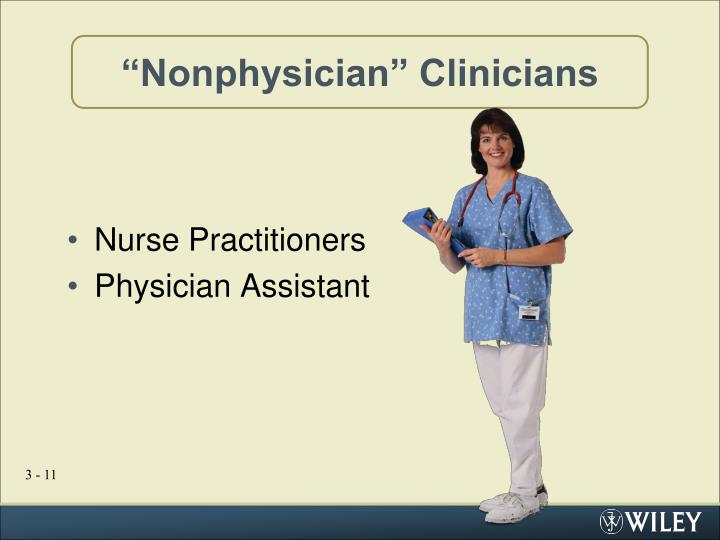The advertisement showcases a female nurse, depicted on the left side of the image, who has medium-length hair with bangs and is wearing blue scrubs, white pants, and white shoes. She has a blue three-ring binder in her hand and a stethoscope around her neck. To her left are bullet points in black ink, stating "Nurse Practitioners" and "Physician Assistant," with “Non-Physician Clinicians” above them in blue ink and quotation marks. At the bottom left, there is "3-11" in black font. The bottom right features the company logo of Wiley, written in white font, along with an upside-down scale. The background is off-white, with a blue border at the bottom.